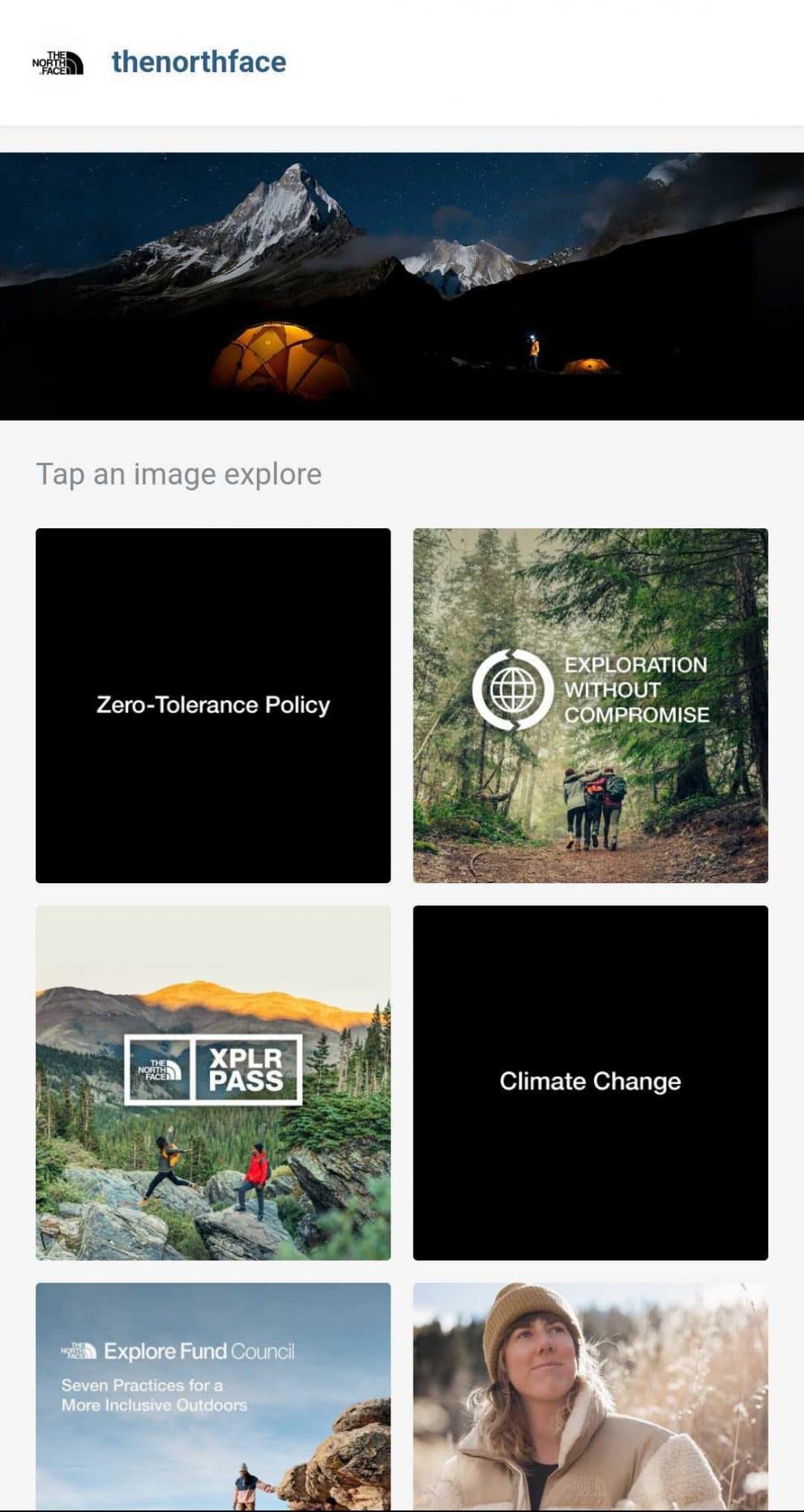The image features the logo of "The North Face" in bold black text. The logo is arranged vertically with the word "The" positioned above "North," which in turn is above "Face." Each word is centrally aligned. To the right of this text, there are three black, curved lines that resemble a tilted and partially chopped Wi-Fi symbol. 

The first black line originates from the "E" in "The" and curves downward to the right. The second black line emerges from the "H" in "North" and also curves downward to the right, following a similar arc to the first line. The third black line starts from the "E" in "Face" and extends outward, but it doesn’t curve as much, appearing more like a short nub. 

Interspersed between these black lines are thin white lines, which enhance the contrast and clarity of the curved design. Additionally, thin white lines are present between the words "The" and "North," as well as between "North" and "Face," maintaining visual separation while contributing to the overall aesthetic of the logo.